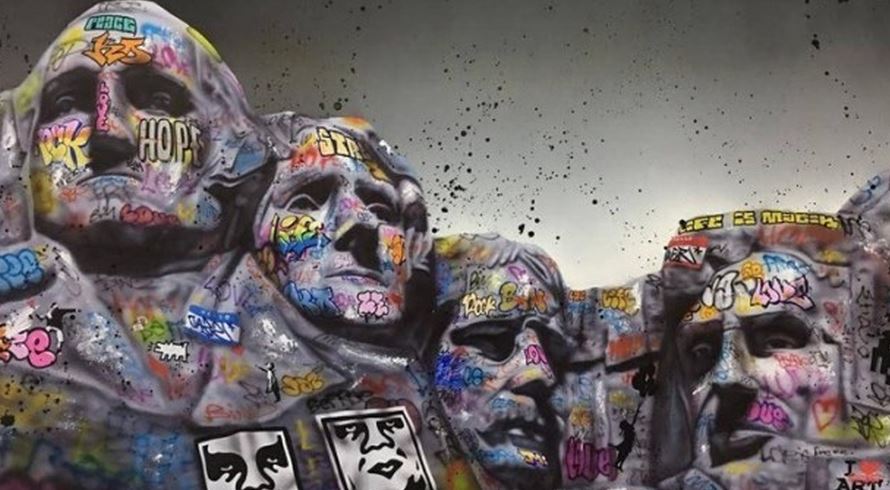This image is a detailed and colorful portrayal of Mount Rushmore with a modern twist. The iconic faces of the four presidents are draped in an array of vibrant graffiti, emphasizing a mix of messages such as "hope," "peace," and other multicolored scribbles in shades of purple, blue, pink, green, and yellow. The graffiti includes airbrush text and various detailed drawings, including a small image of a barking dog and some illustrated faces. The scene is punctuated by two rectangular stickers positioned at the center bottom and an additional text near the lower-right corner stating, "I love art." The background and the statues themselves are largely gray, contributing to a stark contrast between the muted tones of the original sculpture and the vivid graffiti. Dark specks, resembling splattered black paint or falling ash, accentuate the darkened sky and top right area, adding to the grungy, urban feel of this artistic rendition.